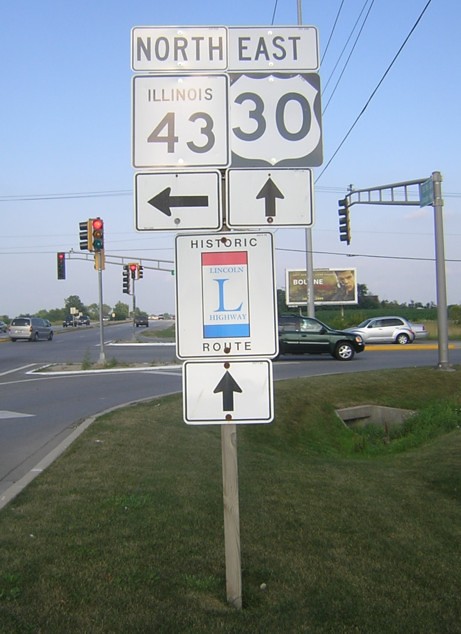This photograph captures a complex array of road signs clustered on a single pole at a busy intersection in Illinois. Dominating the scene, the topmost signs are white with black text and symbols. From left to right, they indicate "North Illinois 43" with a left-pointing arrow and "East Highway 30" with an upward-pointing arrow. Below these, a sign marking the Historic Lincoln Highway features a prominent, large "L" divided by a red top and blue bottom. Another black arrow below this sign also points straight ahead, signaling the direction of the Lincoln Highway. The busy street stretches into the distance with multiple cars and several stoplights visible, some of which display red signals. A road running perpendicular to the main highway is likely North Illinois 43. In the background, a partially obscured billboard with a man's face adds to the urban setting's detail and complexity.